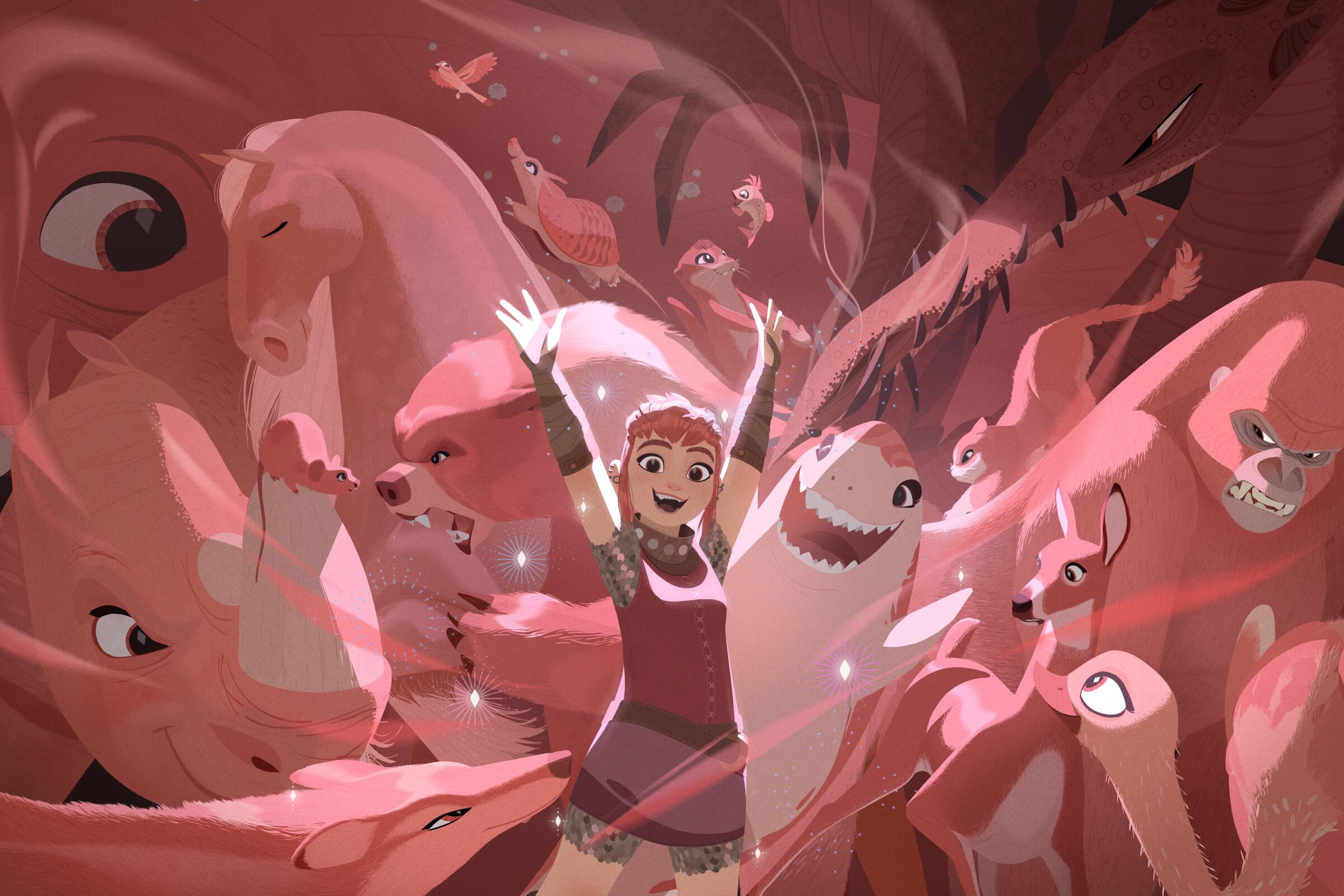This image depicts a vibrant, cartoon-like scene predominantly bathed in pink hues, featuring a multitude of animals seamlessly blending into the background due to their uniform coloration. Centered in the composition is Nimona, a character from the popular film series of the same name. Nimona stands cheerfully with her arms raised above her head, wearing gray gloves, a mauve tank top, and a light purple skirt that matches the overall color scheme. Her pink hair is styled in a bun, and she smiles radiantly with dark eyes. Surrounding her in a harmonious array are various animals such as a unicorn, a rat, a bear, an armadillo, a cat, a gorilla, a deer, a swan or flamingo, a shark, a rhino, a horse, a fox, birds, meerkats, an ostrich, and even does. The entire scene exudes a cohesive, whimsical charm, accentuated by a central beam of light highlighting Nimona and the animals around her, creating a uniquely captivating and clean visual.